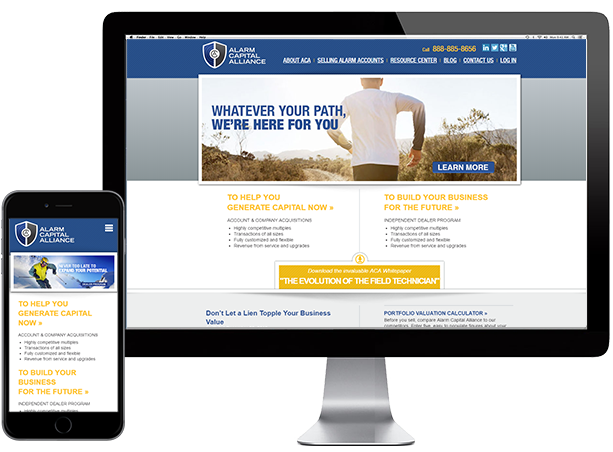The image appears to be a detailed advertisement for Alarm Capital Alliance, featuring various promotional elements laid out across different sections.

On the left side of the image, there's a stylized graphic of a black cell phone displaying a website. The website prominently features the name "Alarm Capital Alliance" in white text. There is a distinctive shield logo that is split into two colors—blue on the left and brown on the right—with a gray circular emblem in the middle. Below the website text, three horizontal white lines are also visible.

Further down, there's an image of a person skiing, dressed in bright neon yellow and blue attire. Accompanying this image is white text overlaying it. Below this, orange and black text reads, "To help you generate capital now," followed by a blurry section of black text that seems unreadable. Additional orange text states, "To build your business for the future."

To the right, there's an image of a desktop monitor that closely resembles an Apple iMac with a thick black bezel and a silver stand. The monitor also displays the website for Alarm Capital Alliance, featuring the same brown and blue shield logo. Below the logo, several white submenu items are listed: "Selling Alarm Accounts," "About ACA," "Resource Center," "Blog," "Contact Us," and "Log in." A gold phone number appears at the top, alongside icons for LinkedIn, Twitter, Google Plus, and another social media platform. Above this, a white bar with black text is visible.

Descending further, another promotional image appears with the text "Navy, whatever your path we're here for you," alongside an image of a man dressed in white jogging. A blue and white box below invites viewers to "Learn More." More gold and black text reads, "To help you generate capital now," and black text again states, "To build your business for the future." A gold and white box at the bottom contains the phrase "The Evolution of the Field Technician," and additional blue text is present at the very bottom of the image.